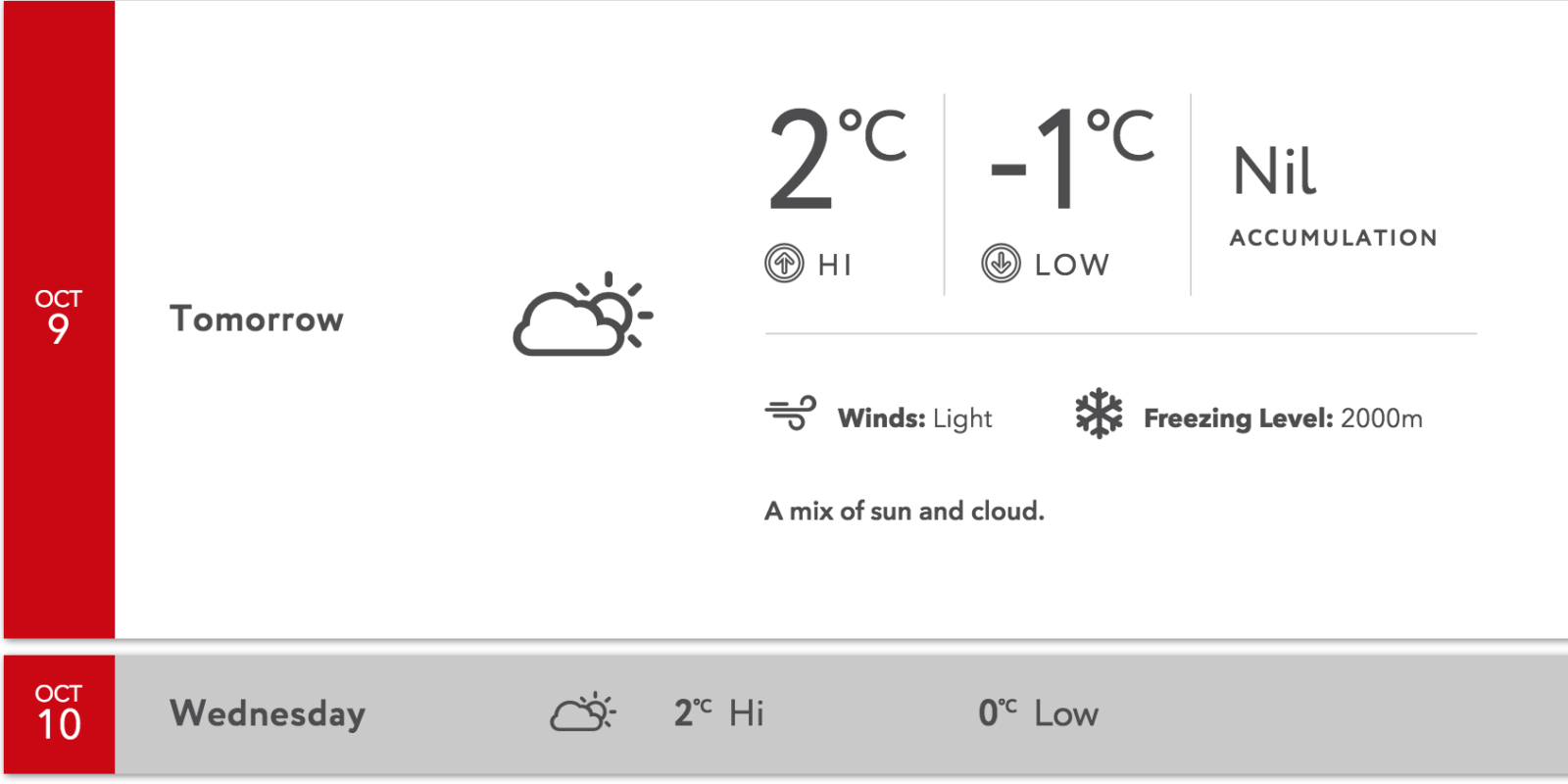In the photographic image, we see a weather forecast in a rectangular box. On the left side of the box, there is a vertical red banner running the length of the box, displaying the date "October 9th." In bold black font, the word "Tomorrow" is prominently featured near the top. Below this, a partly cloudy icon with the sun peeking out of the cloud is shown, indicating the expected weather.

The temperature forecast is displayed in large font: "2°C." Additionally, there are two circles with arrows indicating high and low temperatures, reading "High: 2°C" and "Low: -1°C." The forecast mentions that precipitation accumulation is expected to be nil.

An icon representing wind shows "Winds: Light." A snowflake icon indicates the freezing level, which is forecasted to be at 2,000 meters. The overall weather prediction is for a mix of sun and clouds.

Below this, there is a gray box showing the forecast for "October 10th, Wednesday." Again, the partly cloudy icon with the sun peeking out is shown. The temperature forecast for this day indicates a high of "2°C" and a low of "0°C."